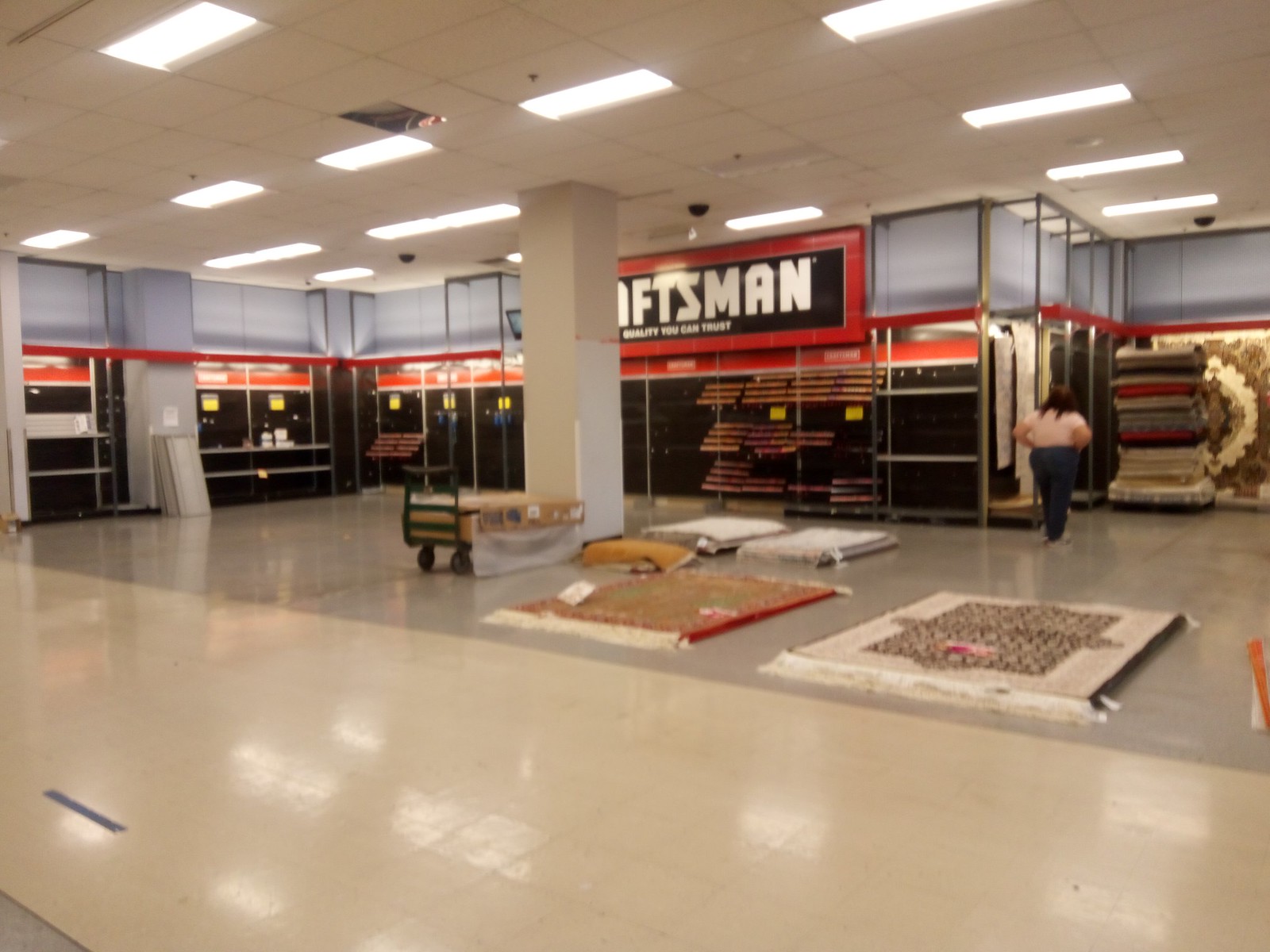This color photograph depicts the interior of a store, possibly a warehouse-type retailer or an outdoor retailer with a section dedicated to Craftsman tools. The store has a large, smooth floor that is tan and gray. In the background, there is a prominent sign partially showing the word "CRAFTSMAN" in large white letters on a black background, bordered by red. Beneath this, in smaller white letters, reads "Quality You Can Trust." A white pole obstructs part of the sign. The shelves, primarily empty and black with red accents, have a few yellow signs.

In the foreground and right-hand side of the image, there are numerous multi-colored rugs piled on the floor and some stacked in the background. The most visible rug near the front is white and blue, and adjacent to it is a red one. There is a woman with dark hair, wearing a white shirt and denim jeans, examining the rugs.

The store ceiling is white with fluorescent lighting, though one ceiling panel seems to be missing. The overall scene gives an impression of a store possibly going out of business or undergoing rearrangement, as many shelves are bare.